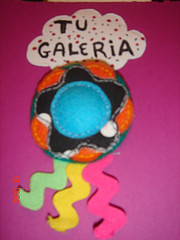The image features a meticulously crafted felt-stuffed design set against a purple background that appears lighter at the center due to the lighting, with the edges transitioning into a darker tone or black. On the left side of the image, a pink watermark with the numbers "191550" runs from top to bottom. The felt creation itself is primarily centered on the image and resembles a circular badge-like structure. The core of this design consists of a blue circle with white stitching, embedded in the middle of a five-pointed, black star that has rounded, beveled edges and white dots along its perimeter. Surrounding the star are additional circles in red and green felt. Three squiggly strands extend downward from the main body of the creation, colored in pink, yellow, and green. At the top of the felt design, a white cloud cutout dotted with red and gray marks can be seen, bearing the text "to Galleria" in black paint.